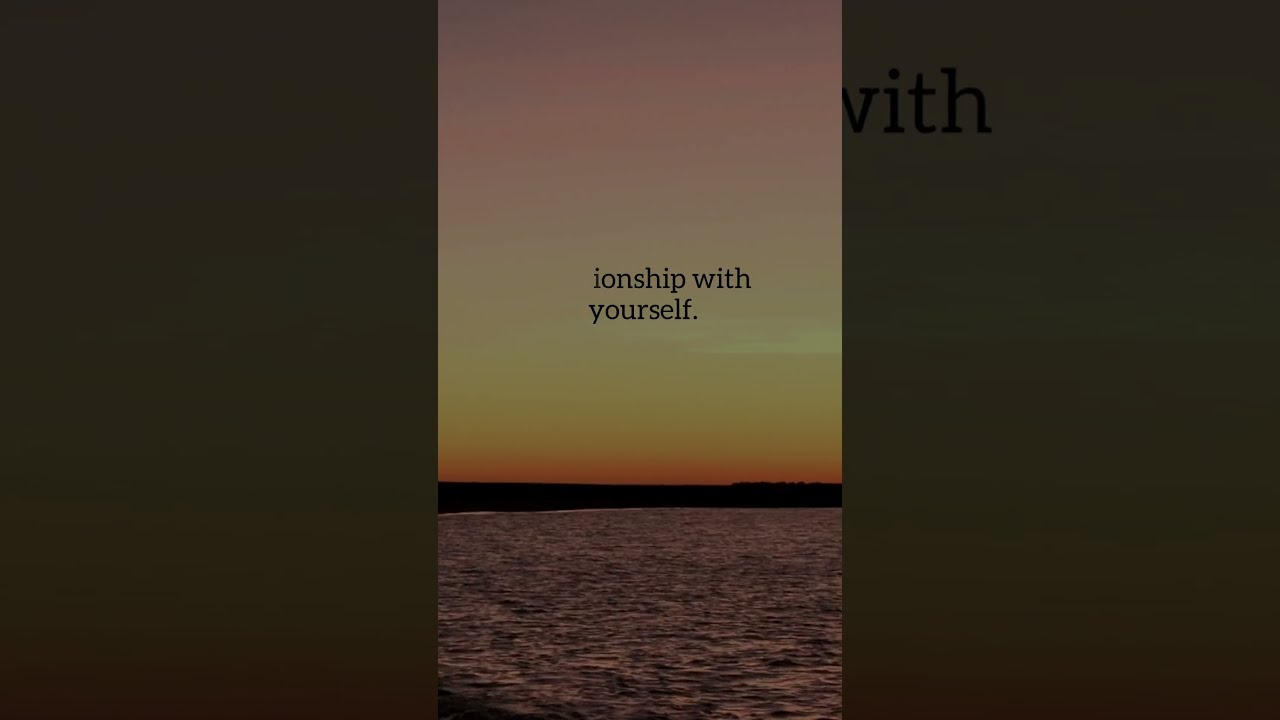The rectangular poster is divided into thirds horizontally, with the outer portions in dark brown or gray. The right side features black lettering at the top, with a partially visible 'W' followed by 'I-T-H.' The central third showcases a stunning twilight scene, a blend of sunset and sunrise hues. The sky transitions from vibrant oranges near the horizon to yellows and creams, fading into light blues and purples, with wisps of pink. A strip of land cuts through the center third, bordered by a rippling body of water extending to the bottom of the poster. Text in black lowercase letters reads "in ship with yourself." The serene water reflects the sky's colors, creating a harmonious blend of light and dark elements. The image evokes the feeling of peering out a window, with the dark blocks on either side framing the calming view outside.